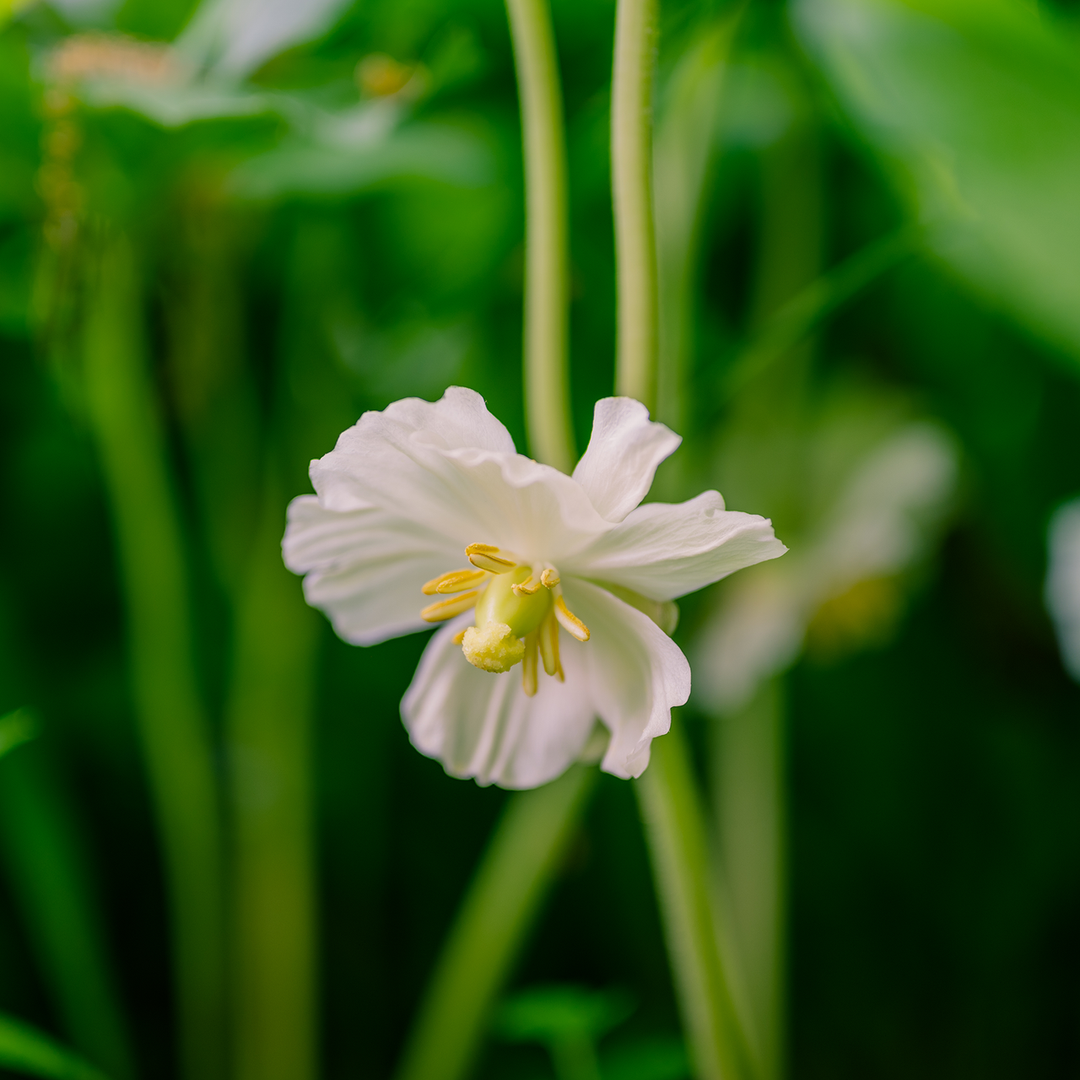This photo is a detailed close-up of a small white flower, which is centrally positioned in the image. The flower features delicate white petals that are gently folded, adding a subtle texture to their appearance. At the heart of the flower is a light yellow center with a slight greenish tint, possibly featuring fine spikes that hint at the flower's pollination mechanism. The backdrop, comprising a lush green landscape of stems, leaves, and possibly other flowers, remains distinctly blurred, emphasizing the crisp and vivid focus on the central white flower. A hint of light pink or orange can be faintly discerned in the upper left of the frame. There is no text, numbers, or other distractions to divert attention from the flower, which stands out sharply against the verdant, out-of-focus background.